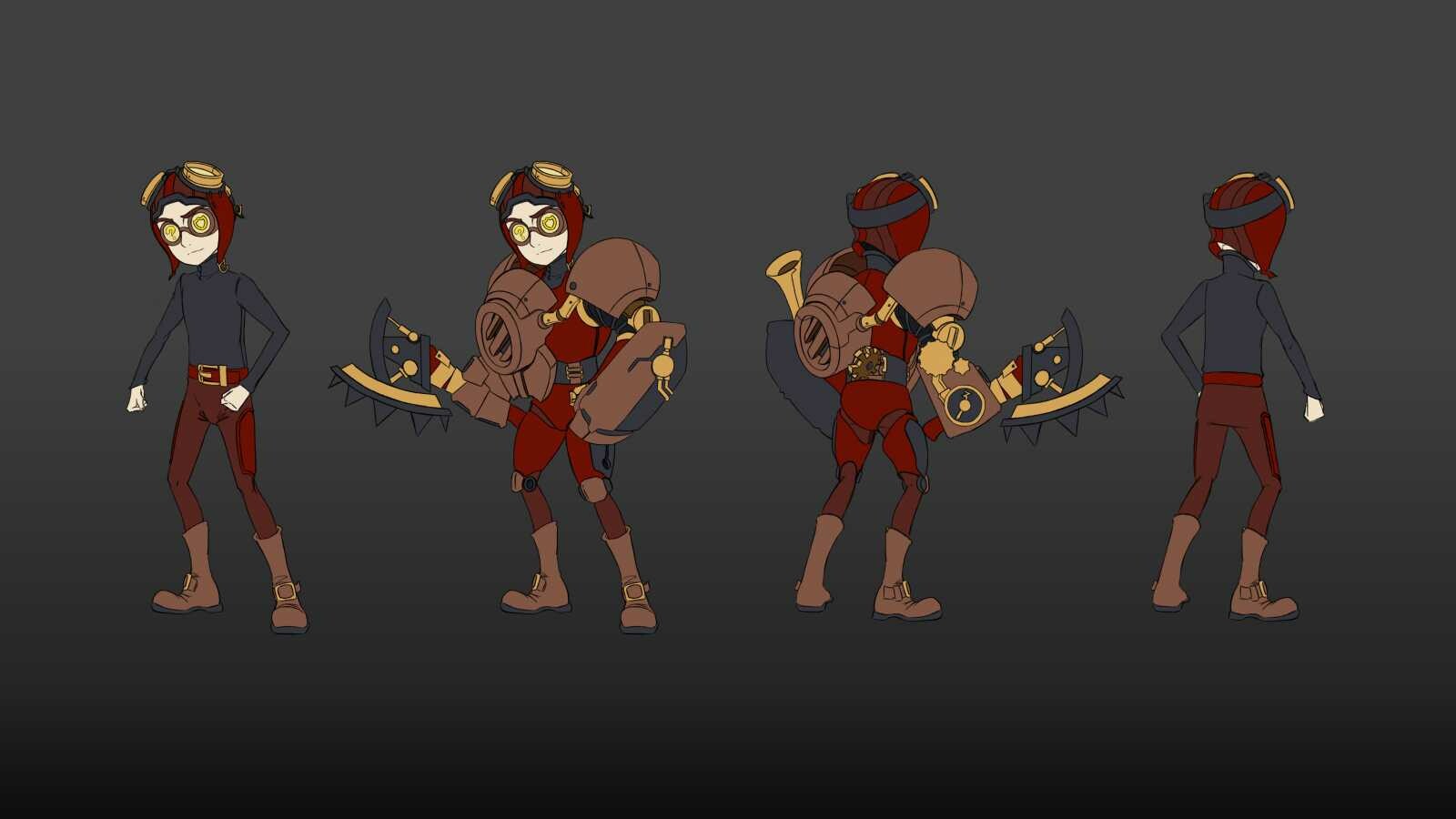The digital illustration features a single cartoon character depicted in four different poses against a gray gradient background that transitions from light at the top to darker at the bottom. The character wears an aviator hat with ear flaps and a set of goggles resting on top, alongside yellow glasses. They sport a gray long-sleeved shirt, brown pants, gray socks, and gray shoes. In the two middle poses, the character is shown with additional exosuit armor on their torso and holding an indiscernible item in their right hand in one of these poses. The character’s facial features and hands are white, and their attire remains consistent across the various stances, alternating only in the presence or absence of the armor.